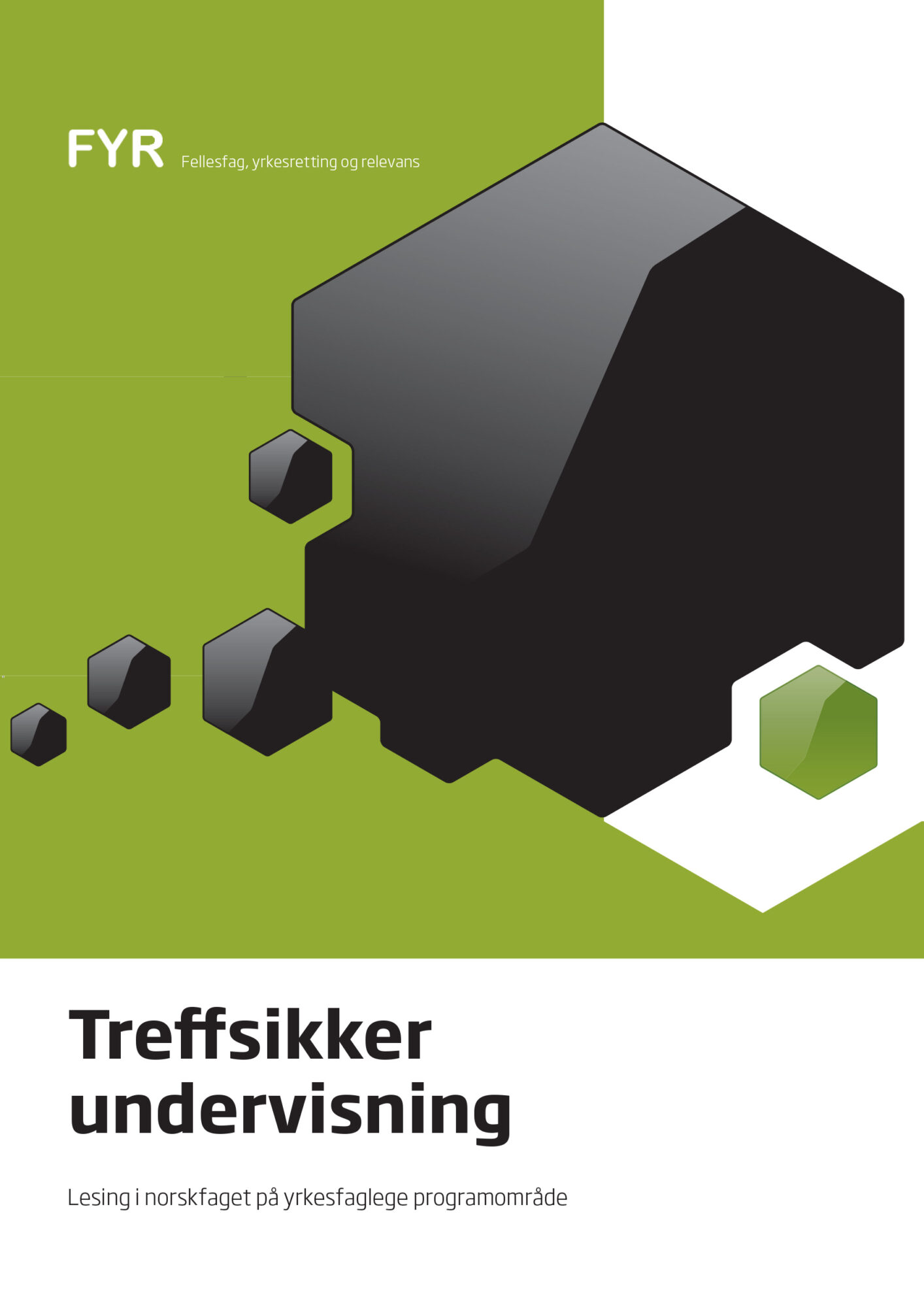The image appears to be an informational card or advertisement. The background is divided into two sections: the left 60% is a darker, swampy green, and the right side is white. In the center of the image, there is a prominent black hexagonal object with a shiny finish, lighter on the upper half and darker on the lower half. This hexagon has smaller hexagonal shapes trailing off to the left, as if parts have broken off from it.

In the upper left corner of the green section, "FYR" is written in white, along with additional white text. Below the central hexagon, on a white background, there are several lines of black text. The first line spells out "T-R-E-F-F-S-I-K-K-E-R" and the second line "U-N-D-E-R-V-I-S-N-I-N-G." Beneath this larger text, there are additional lines of small black text that are difficult to read. The language of the text appears to be Nordic.